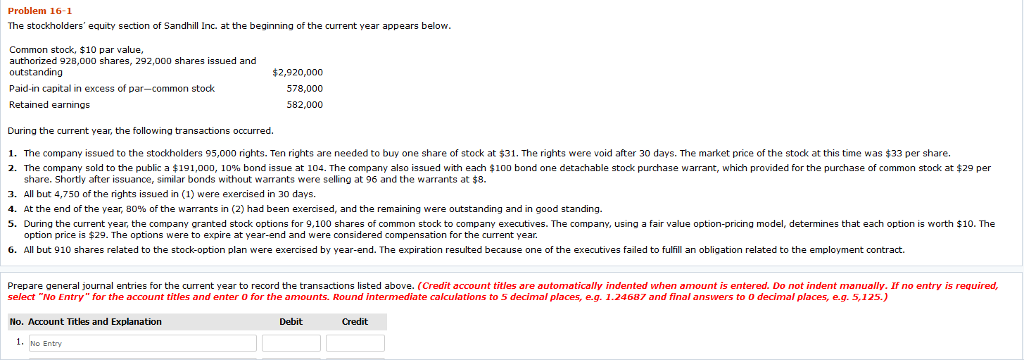This is a detailed caption that describes an informational page, apparently from a computer screen.

---

**Caption:**

The image showcases an informational page appearing to be a digital document. It primarily details financial information related to stockholders' equity for Sandhill Incorporated. At the top of the page, "Problem 16-1" is prominently displayed in red font on the left. Just below, in black letters, it states: "The stockholders' equity section of Sandhill Incorporated at the beginning of the current year appears below."

The document proceeds to provide specific figures related to common stock. It mentions a $10 par value, authorized at 928,000 shares, with 292,000 shares issued and outstanding. It includes details about paid-in capital, excess par for common stock, and retained earnings.

Beneath this, there is an explanatory segment, beginning with: "During the current year, the following transactions occurred." It lists six distinct transactions, which are intended to clarify changes or actions affecting the mentioned financial figures.

Towards the bottom of the page, instructions in black lettering urge the user to prepare journal entries for the current year to record the listed transactions. Additional guidance is presented in red text, emphasizing that credit account titles will automatically indent upon entering an amount; users should not indent manually. It also notes that if no entry is required for a transaction, users should select "No Entry" for the account titles and enter zero for the amounts. A final note instructs to round intermediate calculations to five decimal places.

--- 

This caption aims to provide a comprehensive and clear description of the informational page.